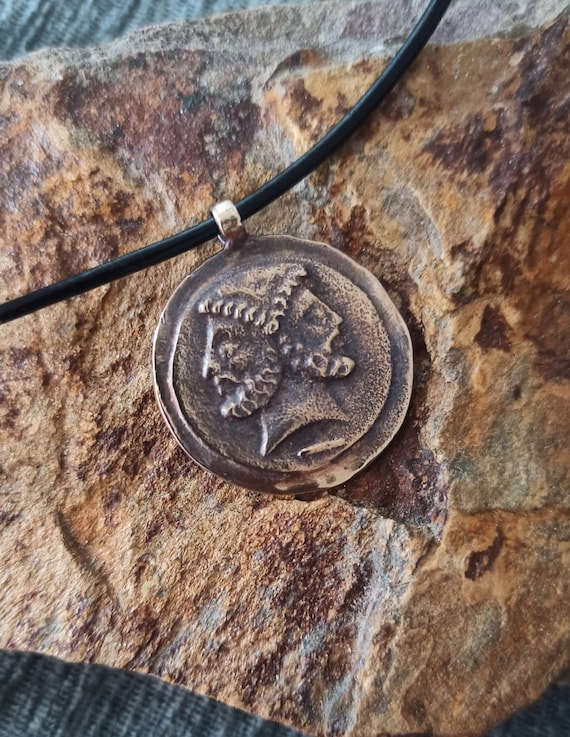This image features a rustic, antique-style necklace with a black cord and a distinctive coin pendant. The coin, appearing old and worn with various nicks and discoloration, prominently displays the two-headed Roman god Janus. The detailed faces, both in silhouette, are oriented in opposite directions—one facing left and the other right—each sharing a single neck. The left face is slightly larger than the right, both depicting a man with a heavy beard and elaborate garments. The pendant is predominantly light and dark brown, complementing the multicolored, textured rock it rests upon. The rock showcases shades of orange, white, and dark brown, adding an earthy backdrop to the display. Beneath the rock, a gray garment subtly peeks through, further enhancing the antique aesthetic of the photograph.